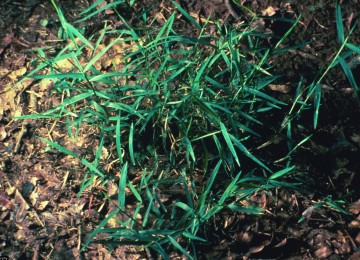This is a detailed close-up photograph of a patch of crabgrass taken from overhead. The lush, dark green blades of grass dominate the center of the image. The background consists mostly of dark brown dirt and wood-like mulch, creating a stark contrast with the greenery. The left-hand side of the photo is slightly lighter, possibly due to lighting, gradually darkening towards the right-hand side, suggesting a shadow. Amidst the grass and mulch, there are some scattered dead leaves and hints of yellowing possibly influenced by the light. Notably, a small hole, about the size of a silver dollar, is partially visible under the grass, potentially indicative of some kind of animal burrow. The overall composition is tightly focused, limiting the view to just this central patch and a few inches of the surrounding mulch.